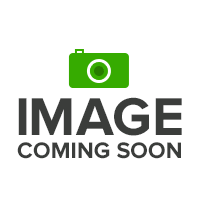The image depicts a nearly full gallon jug of soy sauce positioned on a stainless steel surface, suggesting a commercial kitchen setting. The translucent plastic jug has a white cap and a handle integrated into its side. Inside, the dark soy sauce rises to just a couple of inches below the top. The jug features a white label at its center, showcasing various details: in the middle, Chinese characters 醬油 (zhāngyǒu) indicating "soy sauce", followed by the English words "Soy Sauce" within an orange band. Above this band is an illustration of a bowl with a utensil. The label also displays "all-purpose" and the brand "Regal Foods" along with the net weight of one gallon. Scattered on the label are elements such as a UPC code on both the bottom left and bottom right, and a nutrition facts panel on the left side. Beside the jug sits a small white rectangular tray containing some dark, sticky soy sauce, further emphasizing the culinary context. The stainless steel surface extends beyond the jug, with a white square to the left and a white wall forming the backdrop in the upper part of the image.